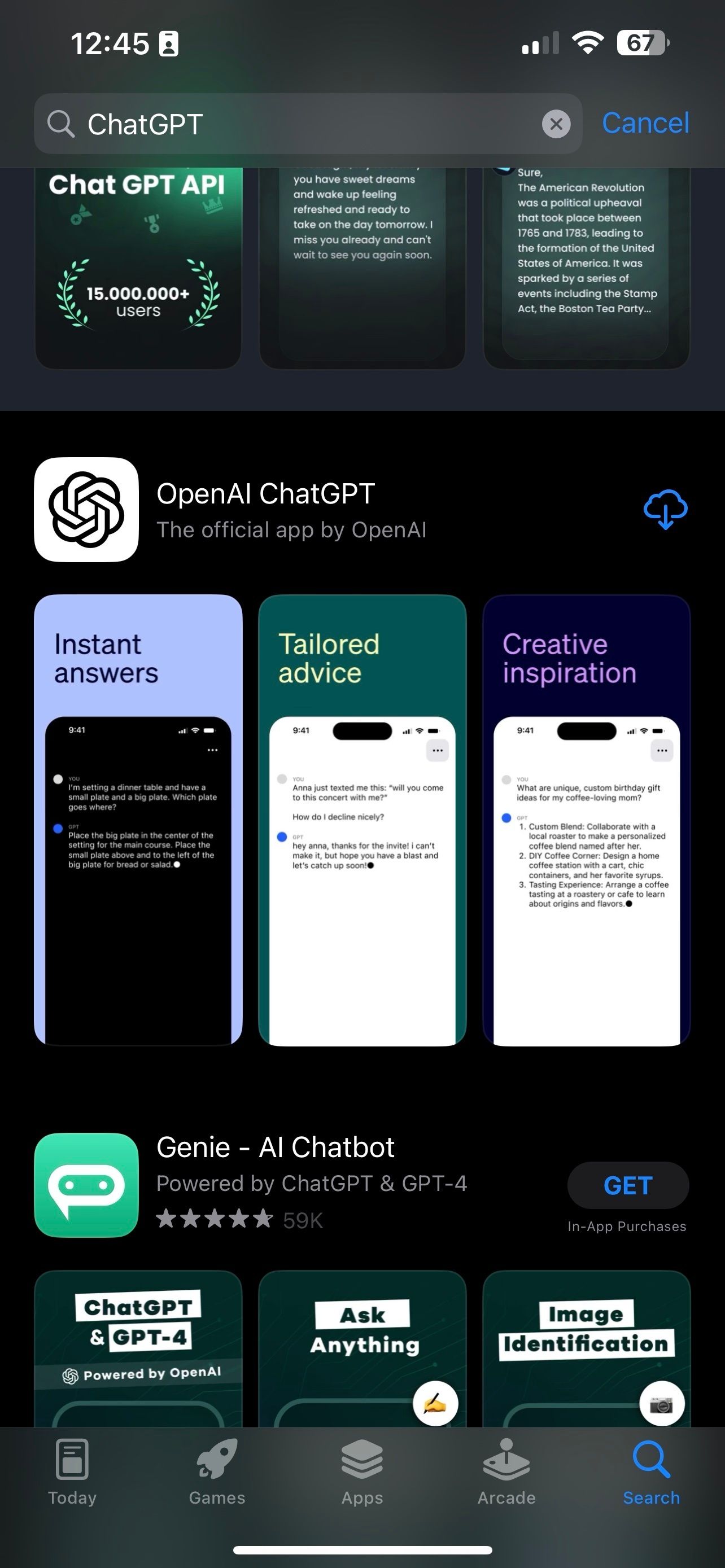The screenshot, captured from a smartphone, displays a search results page in an app store. The search bar at the top of the screen contains the query "chat GPT." The background is predominantly black, with accents of green, teal, blue, and white scattered throughout the interface. At the top of the screen, although the specific app name is obscured, "chat GPT API" stands out as part of the description.

Three app options are prominently listed. The middle selection is "OpenAI ChatGPT," identified as the official app by OpenAI. Its logo features a sophisticated, interwoven braided wreath icon, symbolizing the interconnected nature of advanced AI. At the bottom of the list is an app named "Genie AI Chatbot," distinguished by its teal logo with a white conversation bubble icon containing two dots, indicating a chat interface.